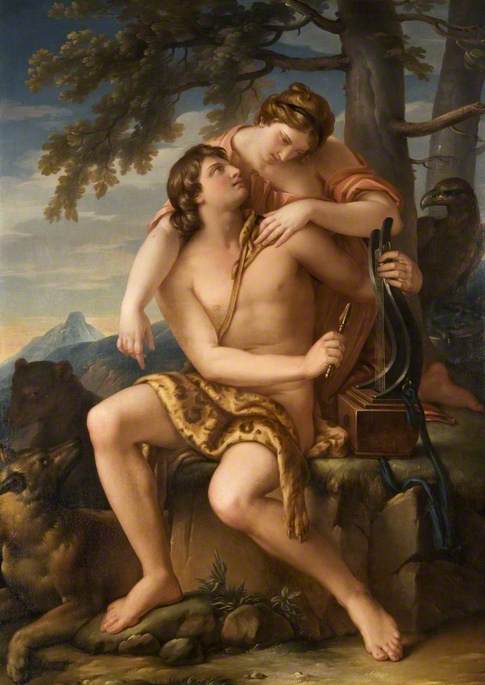The image depicts a detailed painting reminiscent of the Renaissance era, showcasing a natural setting with meticulous attention to elements and figures. At the center, a nearly nude man with medium-length curly hair sits on a rock, his modesty preserved by a draped cloth, possibly green or cheetah print. He holds an arrow in his right hand and places his left hand on a long-handled brown box, possibly a harp. A woman in an orange or pink gown with her hair elegantly pinned up leans over him, gently placing her left hand on his left shoulder and draping her right arm over his right shoulder. The man gazes back at her while she looks towards the harp-like object, suggesting a shared yet individual focus amidst the intimate scene. Behind them, there are trees and a large bird, with mountains in the distance adding to the majestic backdrop. On the left side of the image, two dogs are depicted: one facing away and the other looking back at the man, enhancing the painting's dynamic interaction between the characters and their environment.